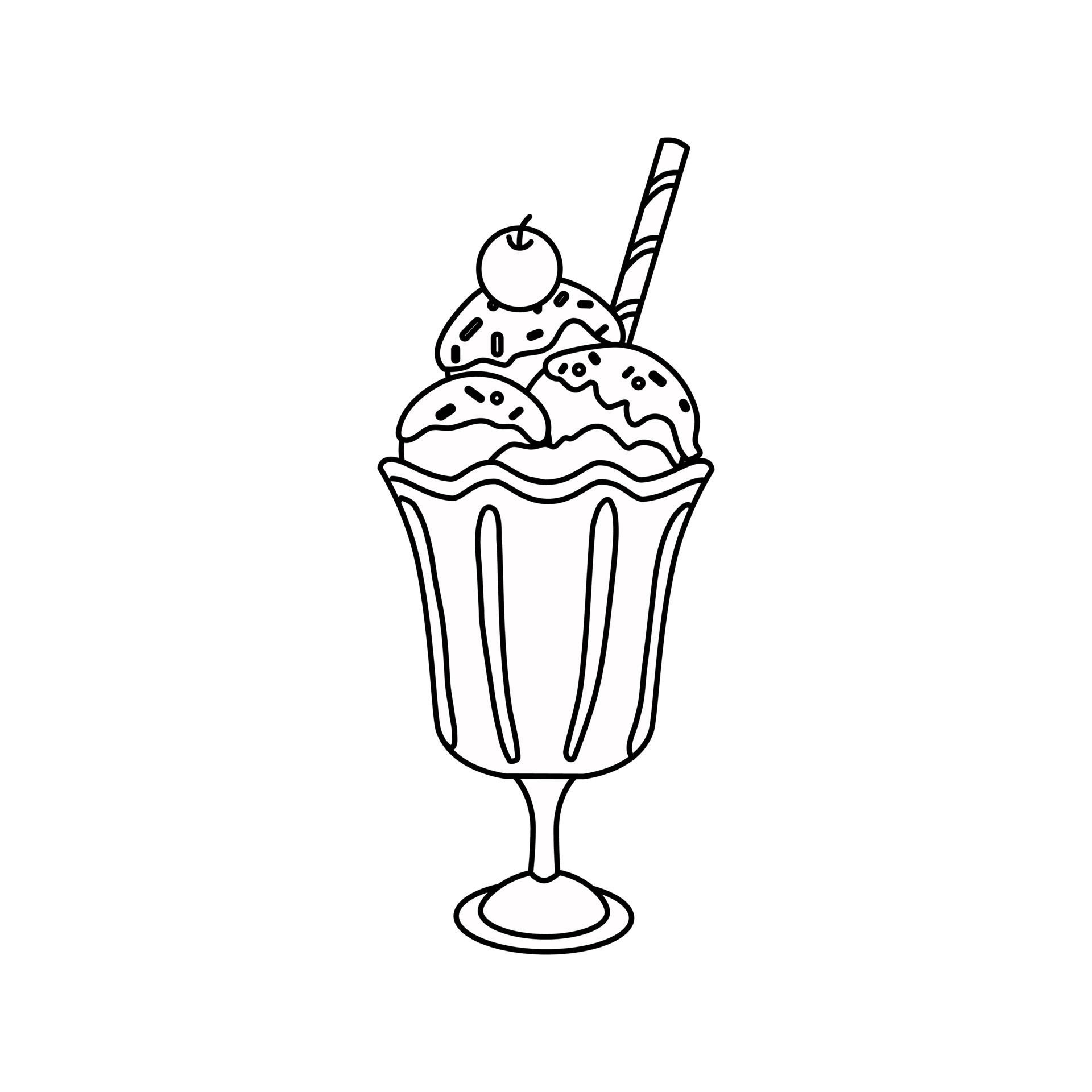This is a detailed, black ink hand-drawn image of an ice cream sundae, devoid of any color and set against a white background, resembling a coloring book illustration. The sundae is presented in a fluted glass, or traditional sundae dish, that resembles a large goblet, complete with a stem and a circular base. The goblet itself is adorned with four distinct divots. The sundae consists of three scoops of ice cream, each topped with what appears to be syrup or sauce and sprinkles. Atop the highest scoop is a cherry, and positioned behind it is a striped straw that wraps around in a clockwise design. The image, completely in black and white, captures the essence of a sweet treat and could easily be used in a coloring book.